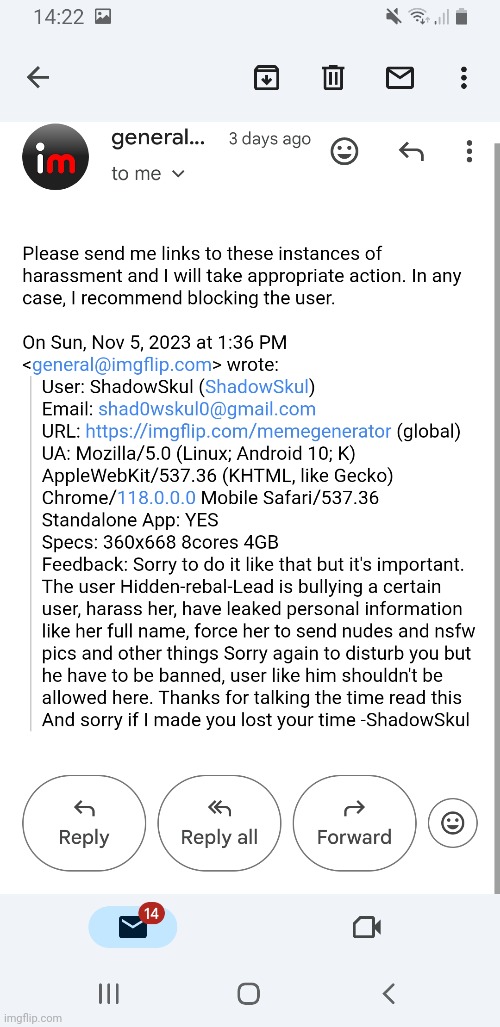This is a detailed caption for an Android device screenshot depicting an email:

---

A screenshot taken on an Android device displays an email received three days ago from a user with a partially visible name starting with "General" followed by three dots. The body of the email reads: "Please send me links to these instances of harassment and I will take appropriate action. In any case, I recommend blocking the user." This email is a response to a previous message the recipient had sent. The initial email’s feedback, visible in the screenshot, says: "Sorry to do it like that, but it's important. The user Hidden Rebel Lead is bullying a certain user, harassing her, having leaked personal information like her full name, forced her to send nudes, and several others. Sorry again to disturb you, but you have to be banned. A user like him shouldn't be allowed here. Thanks for taking the time to read this. Sorry if I made you lost time, Shadow Skull." Additionally, there are 14 other email notifications visible at the bottom of the screen.